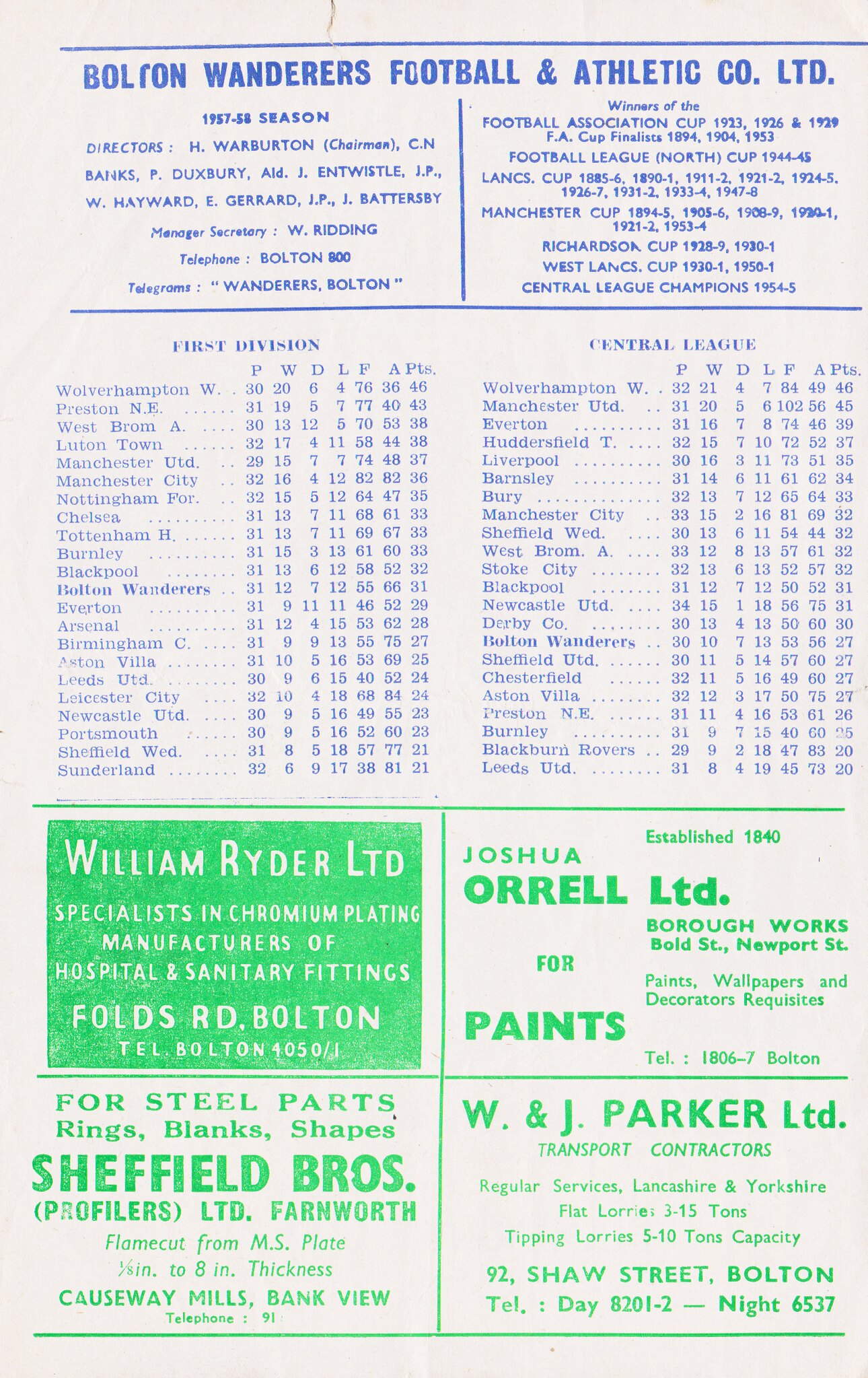The info sheet for a game prominently features the Bolton Wanderers Football and Athletic Co. LTD at the top, highlighting the 1957-58 season and celebrating their victory in the Football Association Cup. The sheet is laid out on a white background with blue headings. The body of the sheet details the "First Division," listing various teams along with their performance stats such as plays, wins, and losses. Parallel to this column is the "Central League" section, also listing different teams and their scores. At the bottom, in neon green text broken into four quadrants, there are advertisements for sponsors. Notably, the sponsors include William Ryder Limited, a specialist in chromium plating and manufacturer of hospital and sanitary fittings; Steel Parks, Riggs, Blanks, Sheffield Brothers; Joshua Orwell Paints; and W.J. Parker Limited Transport Contractors.